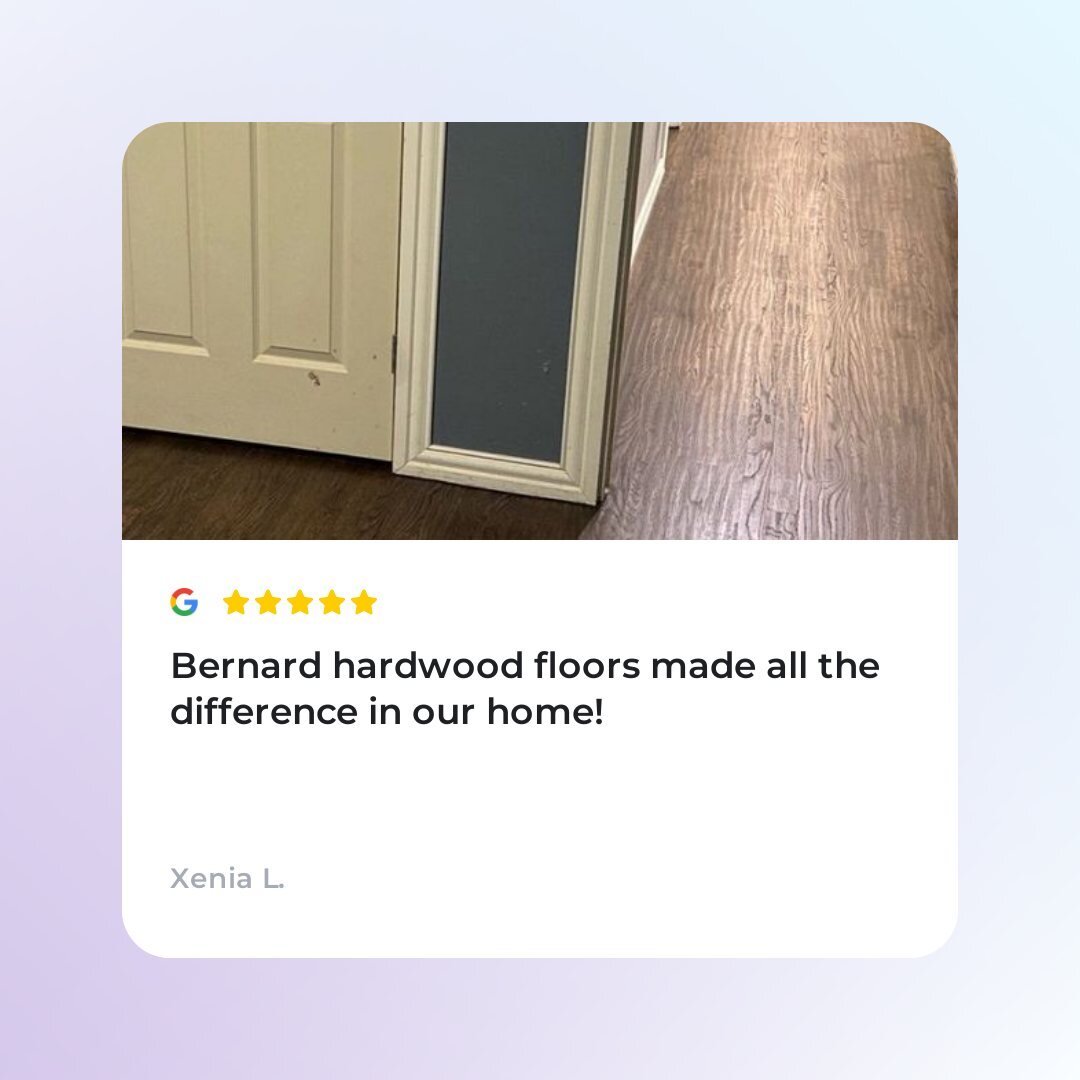In this image, we see a Google Comet advertisement featuring a square, whitish-purple box with hints of blue. Overlaying this background is a second square, which is split into two halves.

The left half contains an image showcasing hardwood floors and a door, emphasizing the elegant and polished look of the flooring. Below this image, the iconic Google 'G' logo is prominently displayed in full color.

To the right of the image, there is a review snippet. It features a row of five golden stars, indicating a top rating. Below the stars, the text reads, "Bernard hardwood floors made all the difference in our home!" in a bold, readable font.

The reviewer is identified below the text as "Zinnia L.," displayed in a distinctive font against a clean, white background. 

Overall, the advertisement effectively highlights the positive impact of Bernard hardwood floors, endorsed by a satisfied customer.